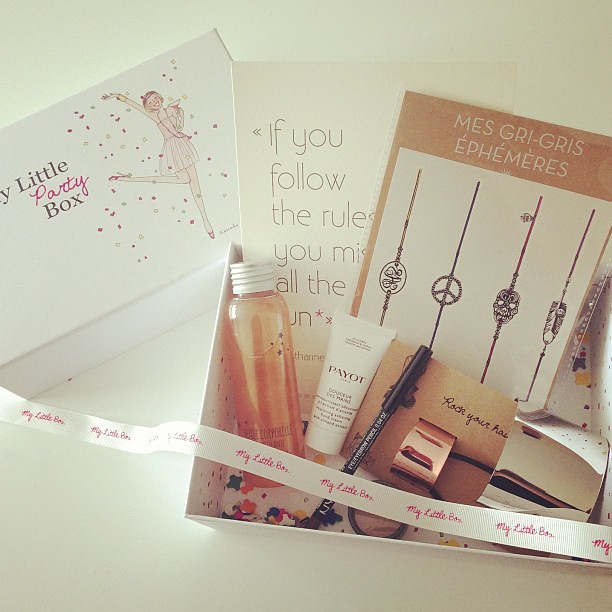The image features a detailed, full-color photograph of an open delivery box brimming with a variety of beauty supplies. Resting on a pristine white table, the box displays both its intriguing contents and a vividly designed lid placed to the bottom left of the box. The lid, adorned with the phrase "My Little Party Box," showcases a cheerful cartoon graphic of a woman in a short pink dress. She is depicted balancing on one leg, merrily holding a margarita glass filled with pink liquid, and surrounded by a festive scattering of pink, yellow, white, and purple confetti.

Inside the box, various beauty products are neatly arranged. Among the visible items are a plastic bottle with a white screw cap, a white tube labeled "Peyote," and a pencil, assumed to be an eyeliner. Additionally, there's a mix of letters or notes and a makeup brush, along with a ribbon that drapes across the box's contents. Adding to the celebratory theme, there's a sign inside the box with the playful message, "If you follow the rules, you miss all the fun," possibly accompanied by some French text. This inviting and fun setting suggests the box is a thoughtfully curated gift set, rich with beauty and hygiene products designed to delight the recipient.